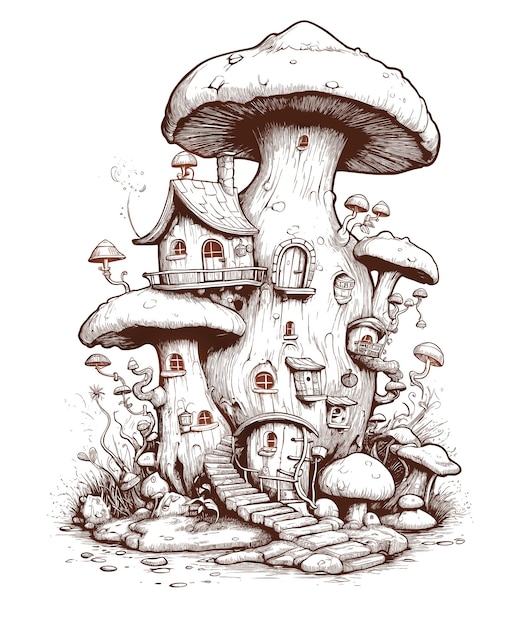The image depicts a detailed drawing of a whimsical mushroom house situated against a white background. Central to the image is an imposing, tall mushroom with a large cap forming the roof of the primary structure. This central mushroom house is adorned with numerous windows and doors, giving it the appearance of a lived-in fairy tale abode. Stairs lead up to a main doorway, suggesting an inviting entrance. Surrounding the main mushroom are smaller mushrooms, each integrated with windows and tiny platforms. One notable smaller house, separate from the mushrooms, is situated to the side and features a traditional roof and chimney. Additionally, small mushrooms sprout from the stems and tops of the larger mushrooms, adding to the magical feel of the scene. At the base of the mushrooms, delicate flowers bloom, contributing to the enchanting atmosphere. Hiding beneath a root, there's a little fairy, blending with the environment and enhancing the fairy tale essence of the artwork. The entire scene is rendered in shades of black, white, and gray, creating a striking contrast that emphasizes the fantastical elements of the mushroom houses.